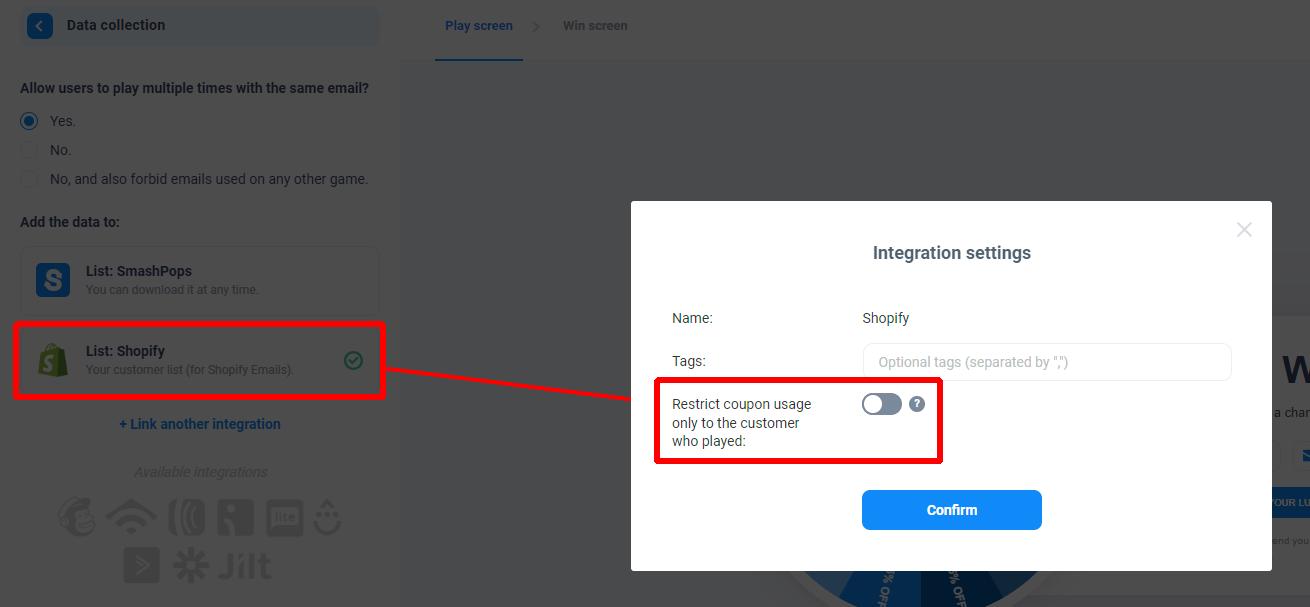The image appears to be a behind-the-scenes look at a web development interface focusing on website integration settings. The background features a black overlay to highlight the main element, a white dialog box with a heading that reads "Integrate Integration Settings". This box includes a close button (X) at the top right.

Inside the white box, there are fields labeled "Name" and "Shopify Tags". An additional input field with faded text indicating, "Optional tags separated by quote marks," is also present. Below these fields, a prominent red box captures attention with the message, "Restrict coupon usage only to customers who play," accompanied by a toggle switch to enable or disable this setting.

Further down, a blue button labeled "Confirm Restrict Coupon Usage" is bordered by a red outline, making it prominent against the overlay. The text next to this button states, "List Shopify your customer list for Shopify emails," indicating integration options that are linked to the website.

Additional sections within the interface are identified as "Play Screen," "Great," and "Win Screen," but no specific details are provided for these options. The overall design suggests a focus on managing integration settings and customer-specific coupon restrictions for a Shopify-linked website.